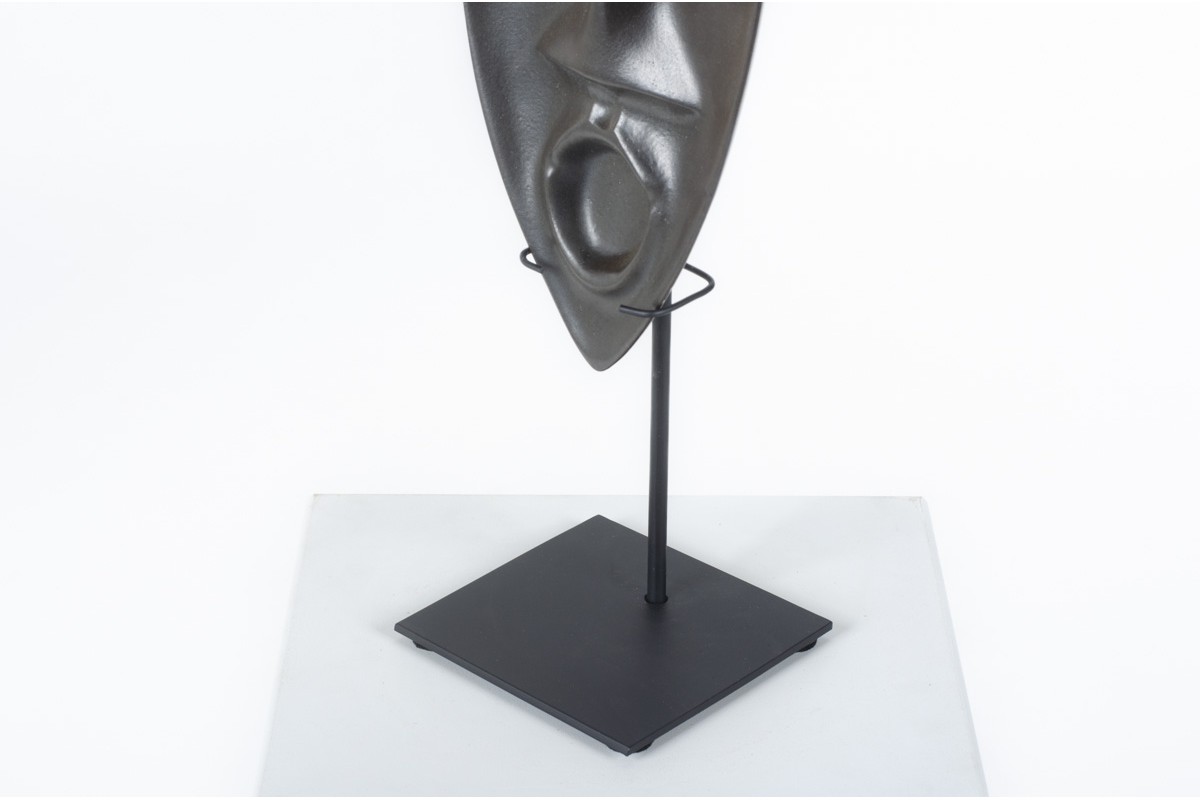This color photograph captures a striking sculpture displayed on a black stand. The stand features a long, black metal holder that extends upwards to secure the art piece. The background is white, possibly a podium or table, accentuating the sculpture. The sculpture itself is a metallic mask in a triangular (or V) shape, with its narrower end at the base, expanding as it rises. The mask prominently features a wide, open mouth, resembling an "O" shape, suggestive of someone yelling or speaking. Additionally, the mask has an indented, pronounced nose that is quite wide and pointed in some descriptions. The artwork, with its expressive facial features, creates a dynamic and somewhat dramatic focal point, accentuated by the stark, supportive stand.